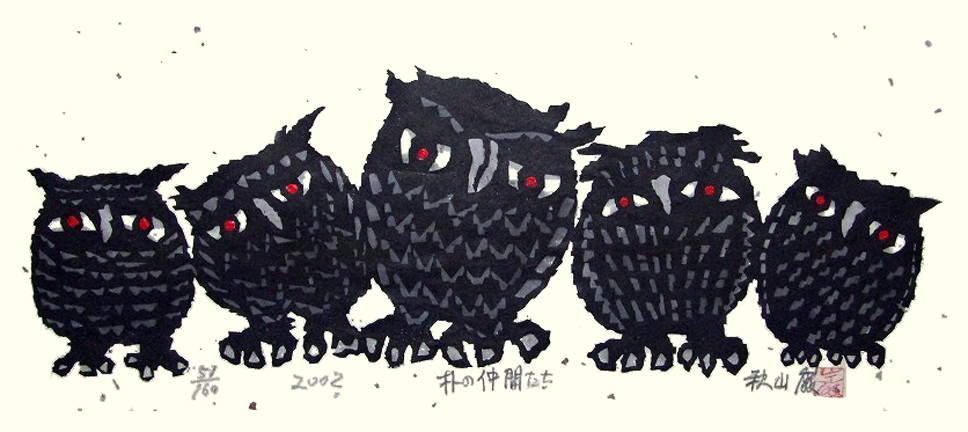The image appears to be a rectangular illustration, likely created using drawing or painting techniques, characterized by a cream or beige background with black speckling. The central focus is on five stylized, cartoonish owls depicted side by side. Each owl is predominantly black with gray markings, including gray noses and three-toed feet with gray toenails. Their eyes are striking, with white irises, black pupils, and red accents, giving them a somewhat menacing appearance. The owls vary slightly in size, with the largest owl in the center and slightly smaller ones flanking it on either side. Below the owls, there is Asian writing, possibly Chinese, along with the numerals '2002' and '51/160,' which could indicate the year of creation and possibly the piece's series number.